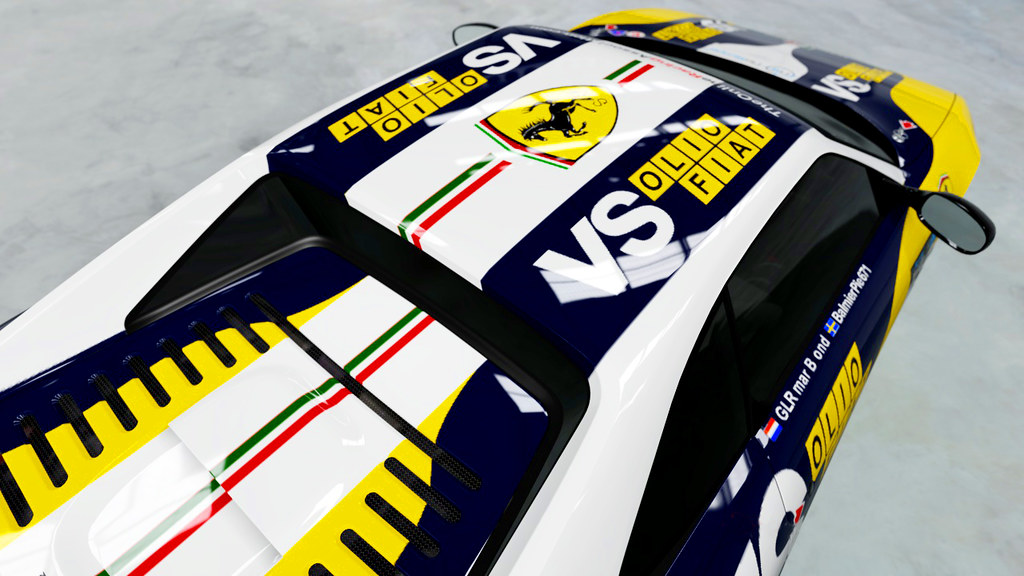The overhead CGI recreation presents a photorealistic image of a racing vehicle, predominantly painted in yellow, black, and white. Atop the roof is a central, upside-down Ferrari logo, featuring a black prancing horse against a yellow shield with a green, white, and red banner above it. The car’s aesthetic is punctuated by stripes of green and red, running vertically from the front windshield to the rear spoiler. Additional detailing includes repetitive logos along the car: the letters "VS" in white set against a blue background, followed by "O-L-I-O" in black within yellow squares, and finally "FIAT" also in black on yellow.

The right side of the car, visible from this overhead angle, reveals deep black windows and a door adorned with the aforementioned logos ("VS," "O-L-I-O," "FIAT"), set against a blue background. This design continuity extends across the hood, which is a vibrant mix of yellow, white, and dark blue, also featuring the same series of logos. The car’s roof and rear spoiler follow suit, their stripes complementing the vehicle's dynamic appearance.

The 3-quarter diagonal angle of the shot places the car’s front to the upper right corner of the frame and its rear toward the lower left. The surrounding environment appears to comprise a marble floor, characterized by light gray, dark gray, and black veined patterns, enhancing the image's realism. The black-framed side view mirror projects out from the right side, contributing to the car’s detailed structure.